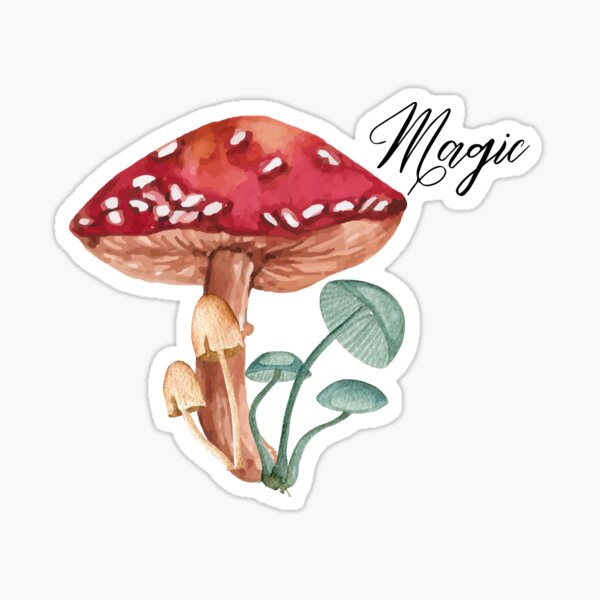The image depicts a vividly detailed colored drawing of a large red mushroom with white spots on its dome. The tan underside and stem of the mushroom add a naturalistic touch to the illustration. Surrounding the main mushroom, there are five smaller mushrooms sprouting from its base: two light tan ones on the left with narrow, helmet-shaped heads and three green ones with large, umbrella-shaped caps on the right. Positioned on a clear white background, the word "MAGIC" is elegantly written in black script to the top right portion of the mushroom's dome. This image appears to be printed on a magnetic strip, possibly used for decorative purposes such as sticking on a refrigerator.